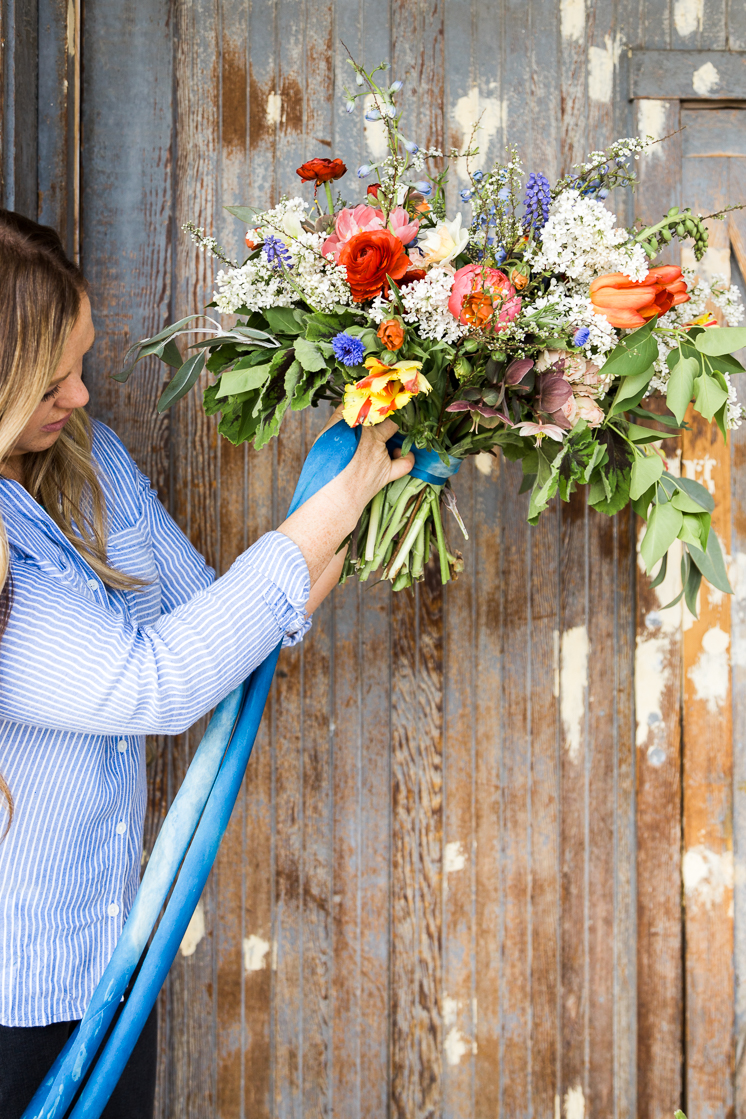In this color photograph, a woman stands in front of a weathered wooden wall that looks like a barn, with a mix of gray and brown hues and sporadic white paint splatters, especially noticeable in the top right and middle right sections. She has long, straight brown hair, cascading down as she faces towards the right side of the image while her body occupies the left middle section. She is dressed in a long-sleeve, collared shirt with blue and white stripes and white buttons, paired with black pants, with her sleeves rolled up for ease.

The woman is meticulously assembling a large, vibrant bouquet of flowers, which she holds prominently in front of her. The blooms in the bouquet display a rich palette of red, blue, orange, and pink, interspersed with green foliage. She is in the process of tying a blue ribbon around the long stems of the bouquet. Despite the clarity on the ribbon, any suggestions of "hoses" seem to be a visual misinterpretation of the ribbon itself as it securely binds the flowers together in her careful hands.